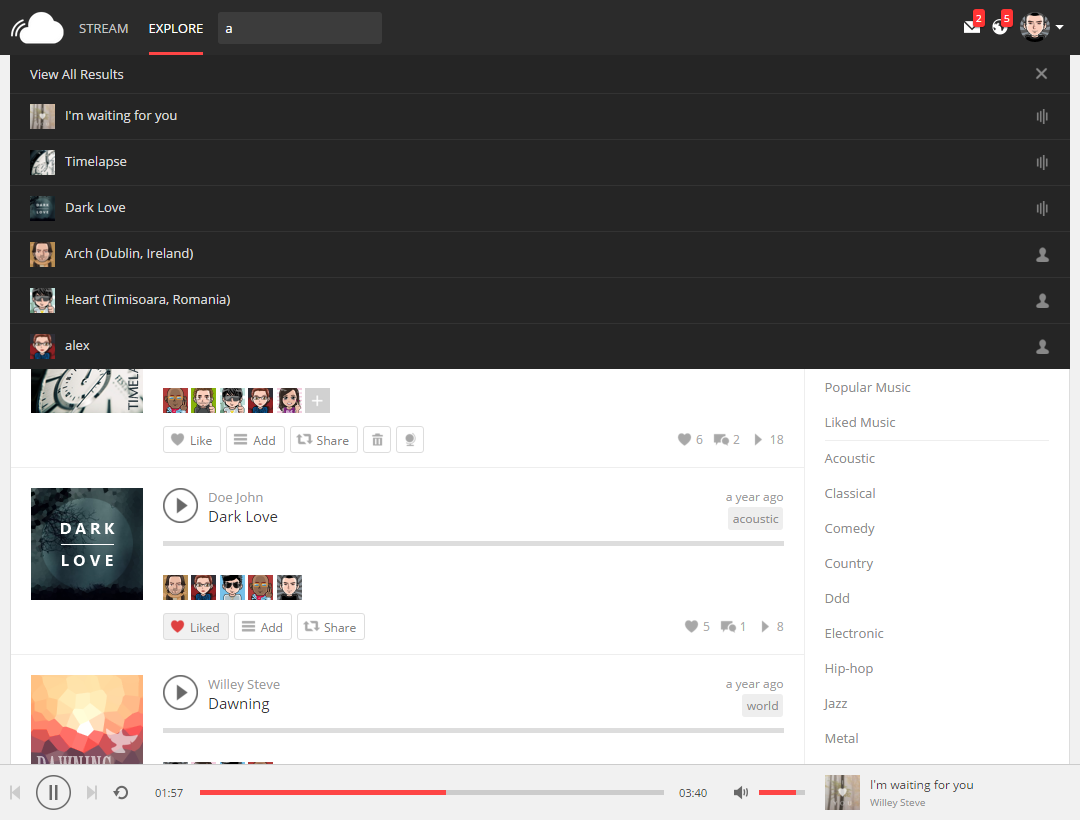The image depicts a music streaming website, likely SoundCloud, judging by the cloud icon emitting sound waves in the upper left-hand corner. In the same area, there are the words "Stream" and "Explore," with "Explore" underlined in red, indicating it is the currently selected tab. The upper right-hand corner features a series of icons: an email icon with a notification badge showing two messages, an earth icon indicating five notifications, and a user profile image resembling a cartoonish male character. Below the "Explore" bar, which contains the letter "A," a message says "View all results," displaying search results including "I'm Waiting for You," "Time Lapse," "Dark Love," "Arch," "Heart," and "Alex."